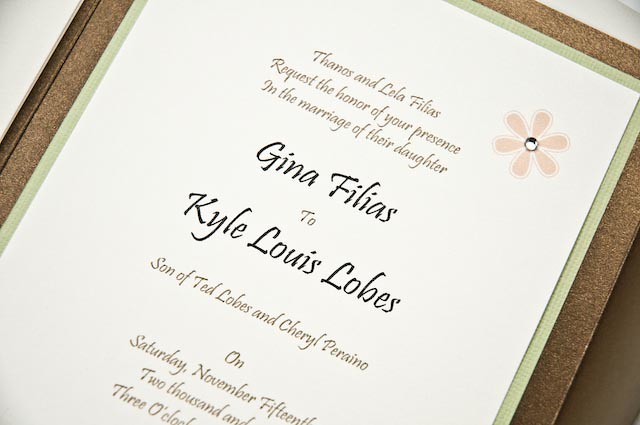The image depicts a high-quality wedding invitation on a slant, showing most of its white-centered body with a distinct decorative border. The invitation's border comprises a brown exterior and a thin green line, followed by a second, inner white border. Prominent within the design, a pink flower with a jewel or gem at its center graces the upper right corner. The text, chiefly displayed in a brown and black script font with some green accents, invites guests to the marriage of Gina Filias, daughter of Thanos and Lila Filias, to Kyle Louis Loebs, son of Ted Loebs and Cheryl Perrino. The largest text highlights the names of the bride and groom. Although the date and time are partially visible, indicating Saturday, November 15th at three o'clock, the precise year remains obscured. The invitation eloquently balances elegance with simplicity, encapsulated by a meticulous layout and detailed embellishments.